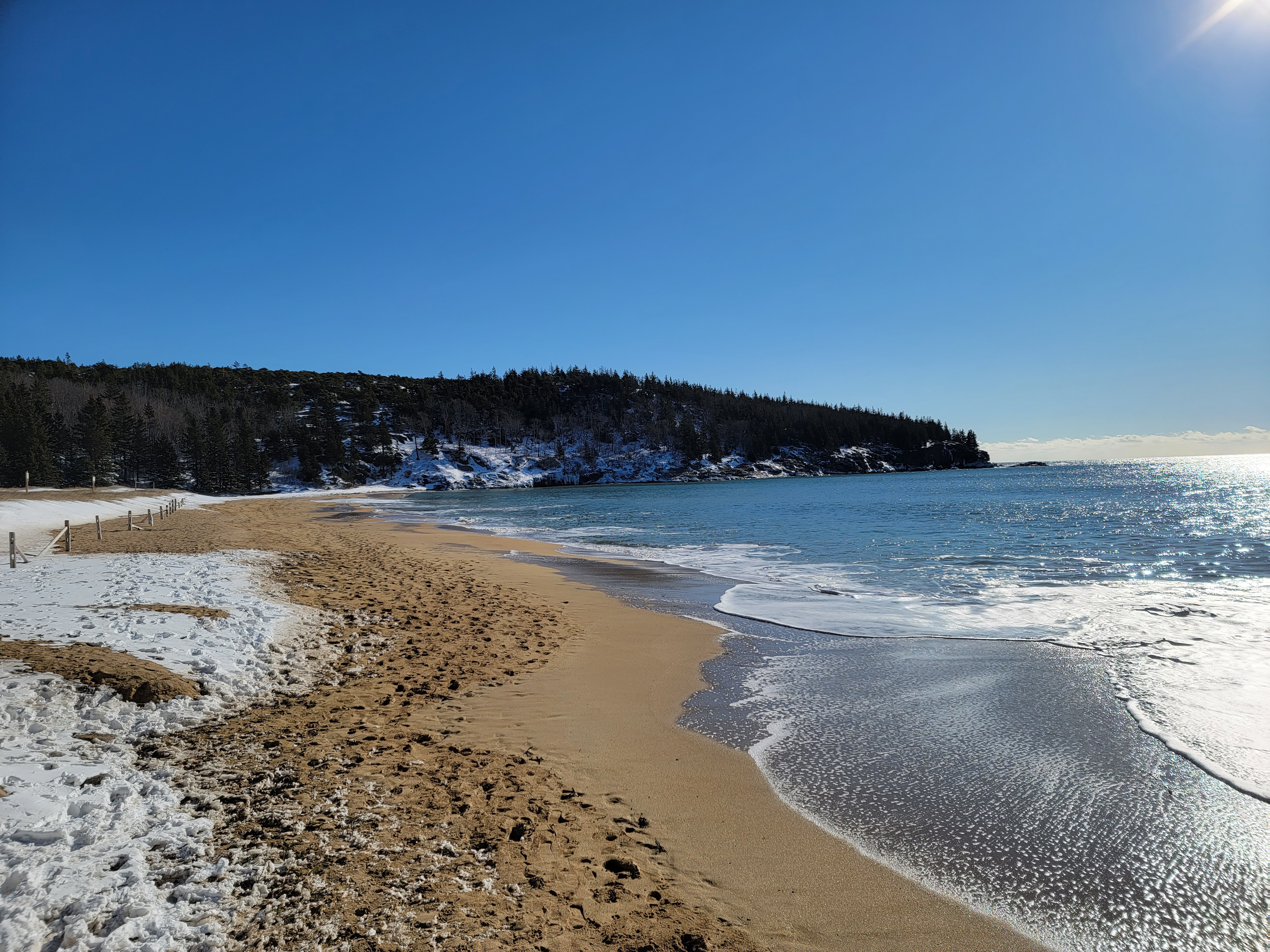The image depicts a serene winter beach scene along the ocean, showcasing a unique blend of sand and snow. The light tan-colored beach appears undisturbed with smooth sand shaped by the lowering tides, creating delicate white foam caps. The shoreline exhibits a jagged pattern where the waves have washed away the snow, blending into the sandy expanse. The ocean itself is a mix of blue and white, suggestive of either cold, frosty waters or the translucence of foam hitting the shore. To the right, the sun, though not visible, casts its rays across the scene. In the background, a hill adorned with dark trees and snow stands tall. The snow rests primarily on the ground, not on the branches. Light clouds also hover near the horizon, adding to the wintry landscape. The beach features wooden fences likely to deter road traffic, with a small road visible in the distance. The sky above is a clear and vibrant blue, creating a picture-perfect day in this northern coastal setting.